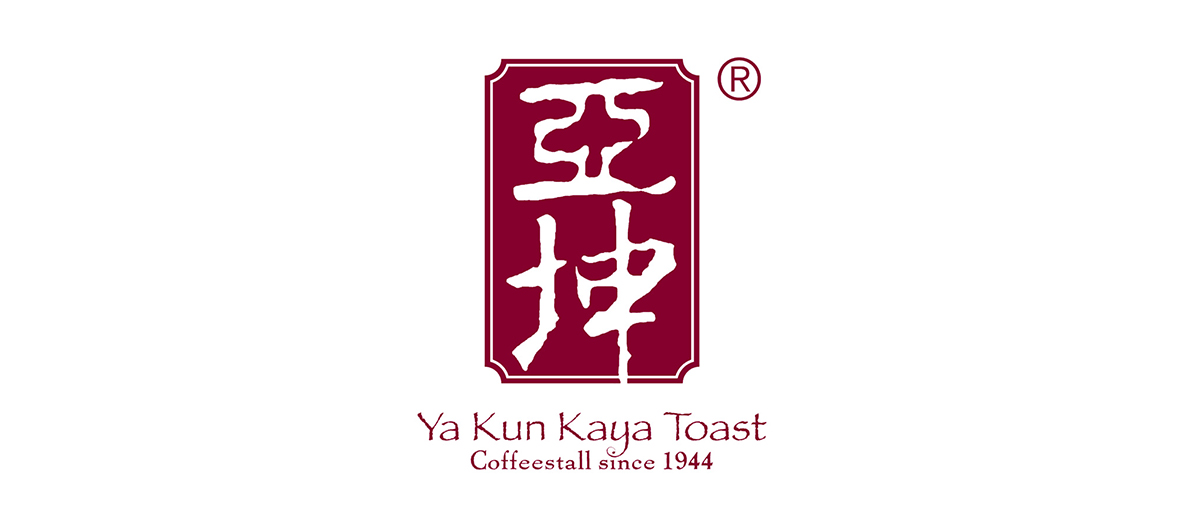This image is of a logo on a white background, featuring a prominent maroon rectangle with indented corners and adorned with a thin white border surrounded by another maroon line. Inside the rectangle, white Chinese symbols are displayed. In the upper right corner of the logo, there is a maroon capital "R" enclosed in a circle, indicating a registered trademark. Below the rectangle, the words "Ya Kun Kaya Toast" are written in maroon, followed by "Coffee Stall since 1944" in the same color, emphasizing the brand's long-standing history.